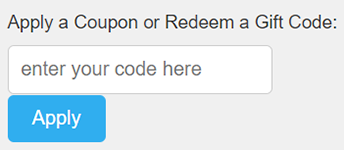The image depicts the coupon code section of a website's checkout process, which is typically found in the payment or order review sections. The background of this section is light gray. At the top of the box, there is black text that reads, "Apply a coupon or redeem a gift code." Below this, there is a white input box with placeholder text that says, "Enter your code here." Beneath the input box, on the left side, is a rounded blue button with white text that says, "Apply." This button is used to apply the entered code to the order.